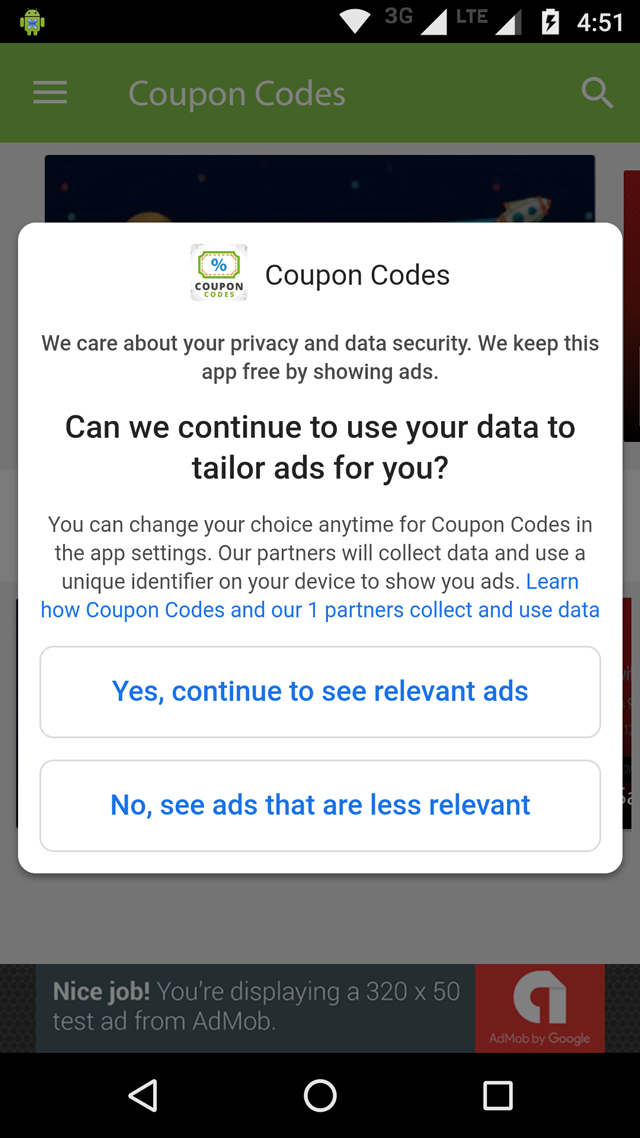This image is a screenshot from the website "Coupon Codes," displaying a privacy and data security notice. The backdrop is a white screen with black and blue text, providing a clear and uncluttered visual experience.

At the very top center of the page is the "Coupon Codes" logo, which consists of a blue percentage sign enclosed within a greenish-yellow square border. To the right of the logo, the site name "Coupon Codes" is prominently displayed in bold text.

The main body of the notice reads: "We care about your privacy and data security. We keep this app free by showing ads. Can we continue to use your data to tailor ads for you? You can change your choice any time for Coupon Codes in the app settings. Our partners will collect data and use a unique identifier on your device to show you ads." This information is written in black text and further emphasizes the site's commitment to user privacy and data security.

Following this section, the text transitions to blue and states: "Learn how Coupon Codes and our partners collect and use data." This indicates an opportunity for users to get more detailed information about data practices.

Below this informative section, there are two actionable options presented as white rectangles bordered in gray. The first button reads "Yes, continue to see relevant ads," providing users with an option to consent to personalized advertisements. The second button, located just below the first, reads "No, see ads that are less relevant," allowing users to opt out of tailored advertising.

This comprehensive notice aims to inform users transparently about the site's data practices and gives them clear choices regarding their consent for personalized advertising.